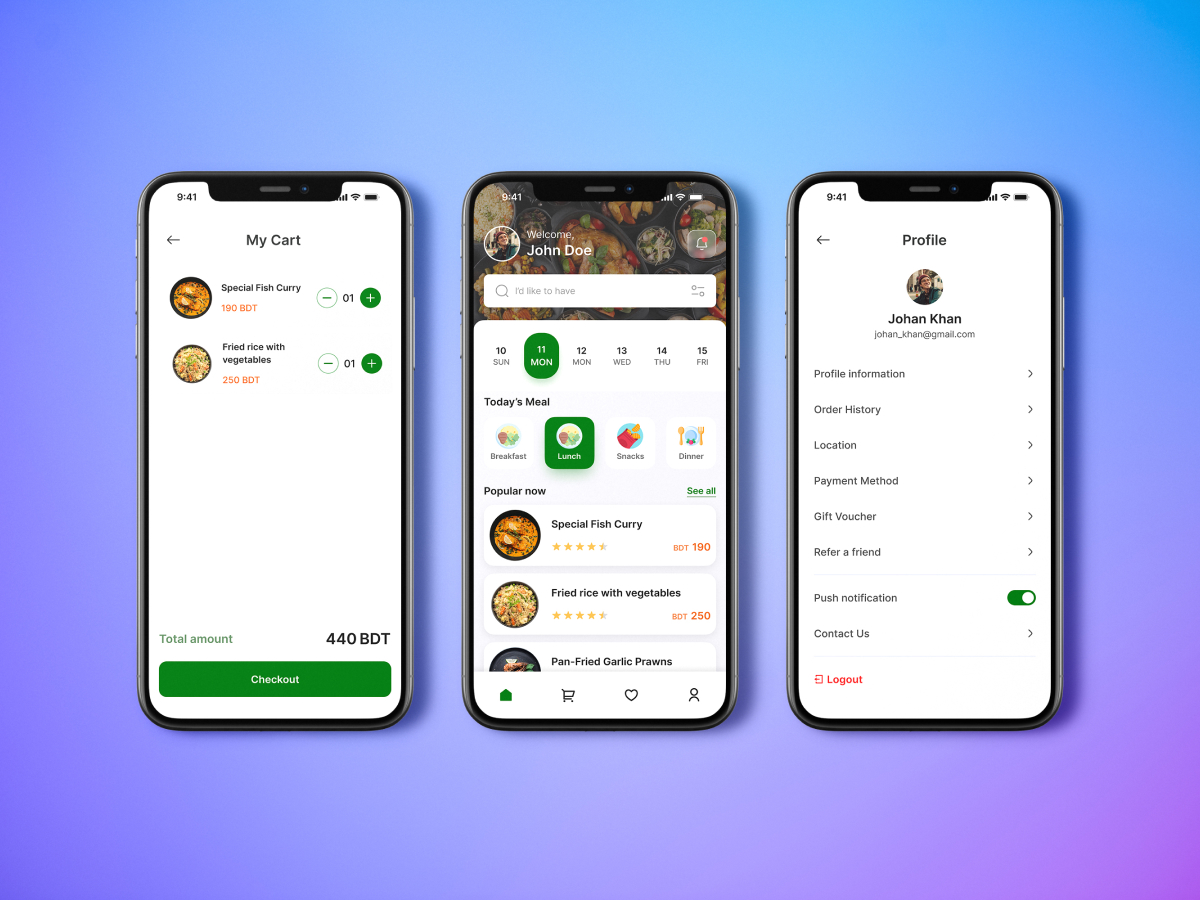A visually striking screenshot displays the interfaces of three distinct smartphones against a gradient background transitioning from blue at the top, through white and gray, to a pinkish purple at the bottom. Each phone screen is captured at precisely the same time, 9:41, with identical battery levels, suggesting the screenshots were taken in quick succession or simultaneously.

In the phone on the left, a cart from a meal planning website is visible. The cart contains two items: "Special Fish Curry," priced at 190 BDT, and "Fried Rice with Vegetables," priced at 250 BDT, totaling 440 BDT.

The middle phone's screen prominently displays the user's name, "John Doe," with a calendar positioned below it, indicating a scheduling or planning app.

The phone on the right shows a profile page where the user is likely able to edit their profile details and settings. This detailed display provides a comprehensive glance into different functionalities and user interfaces within the smartphone environment.